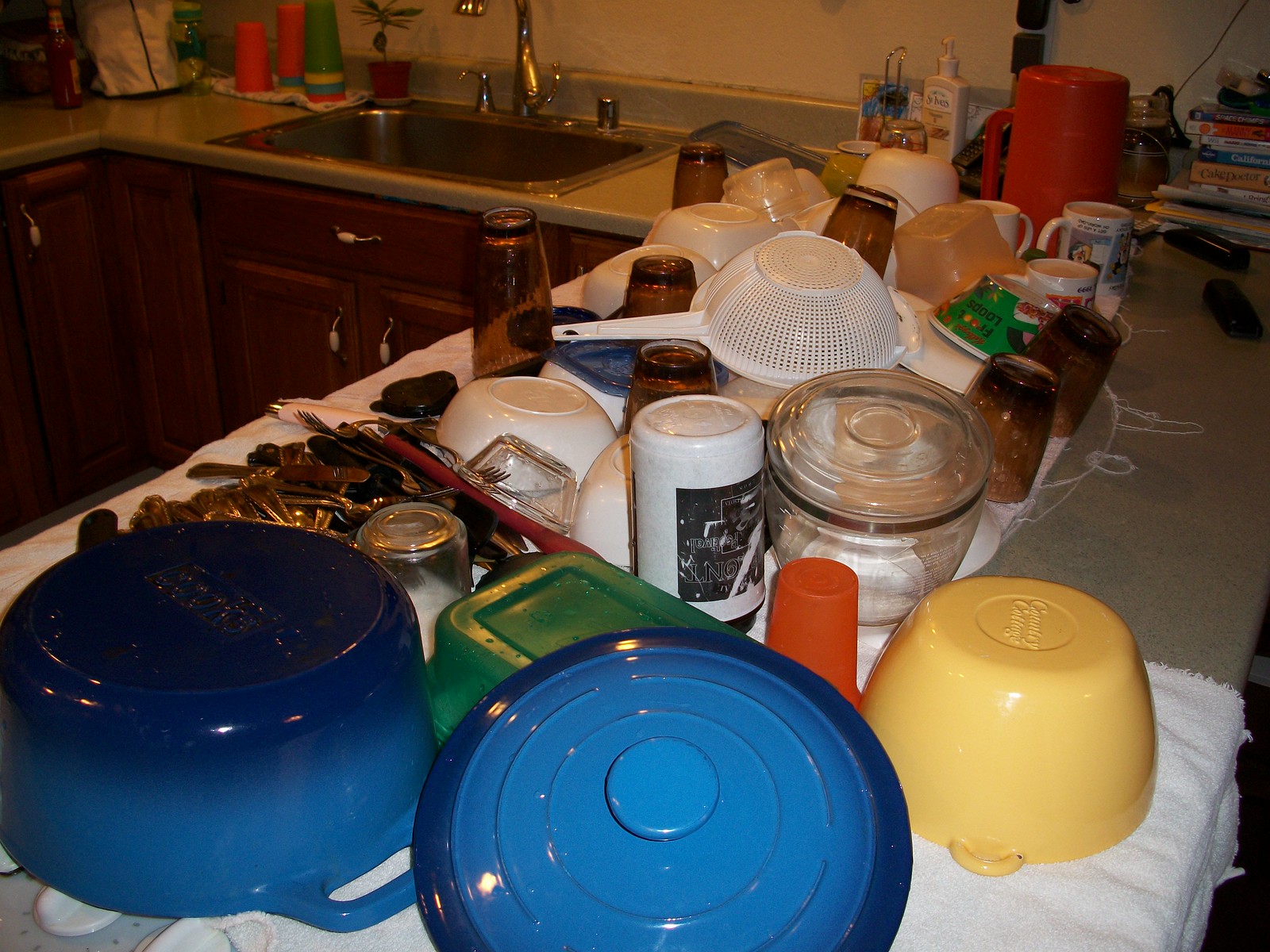This image captures a bustling kitchen scene, showcasing a well-used yet organized space. The background features medium brown, stained cabinets adorned with sleek white and metal drawer pulls and handles. The countertops, forming a practical U-shape, are a light grayish-tan color that complements the white backsplash above them. Centered above the counter is a modern chrome sink faucet. 

In the forefront, an array of clean dishes is neatly piled up, including a notable blue Dutch oven, a bright yellow bowl, and a vivid green pan. Among these are various pieces of silverware, a colander, a versatile coffee pot, a selection of mugs, and some brown glasses. To the left of the sink, a collection of colorful plastic cups can be seen alongside a bottle of sauce. To the right, a bottle of hand lotion is placed near an orange pitcher, commonly used for making lemonade. Additionally, a stack of books is partially visible on the far right, just off the edge of the frame. The entire scene exudes a sense of activity and practical organization, indicative of a space frequently used for cooking and gathering.